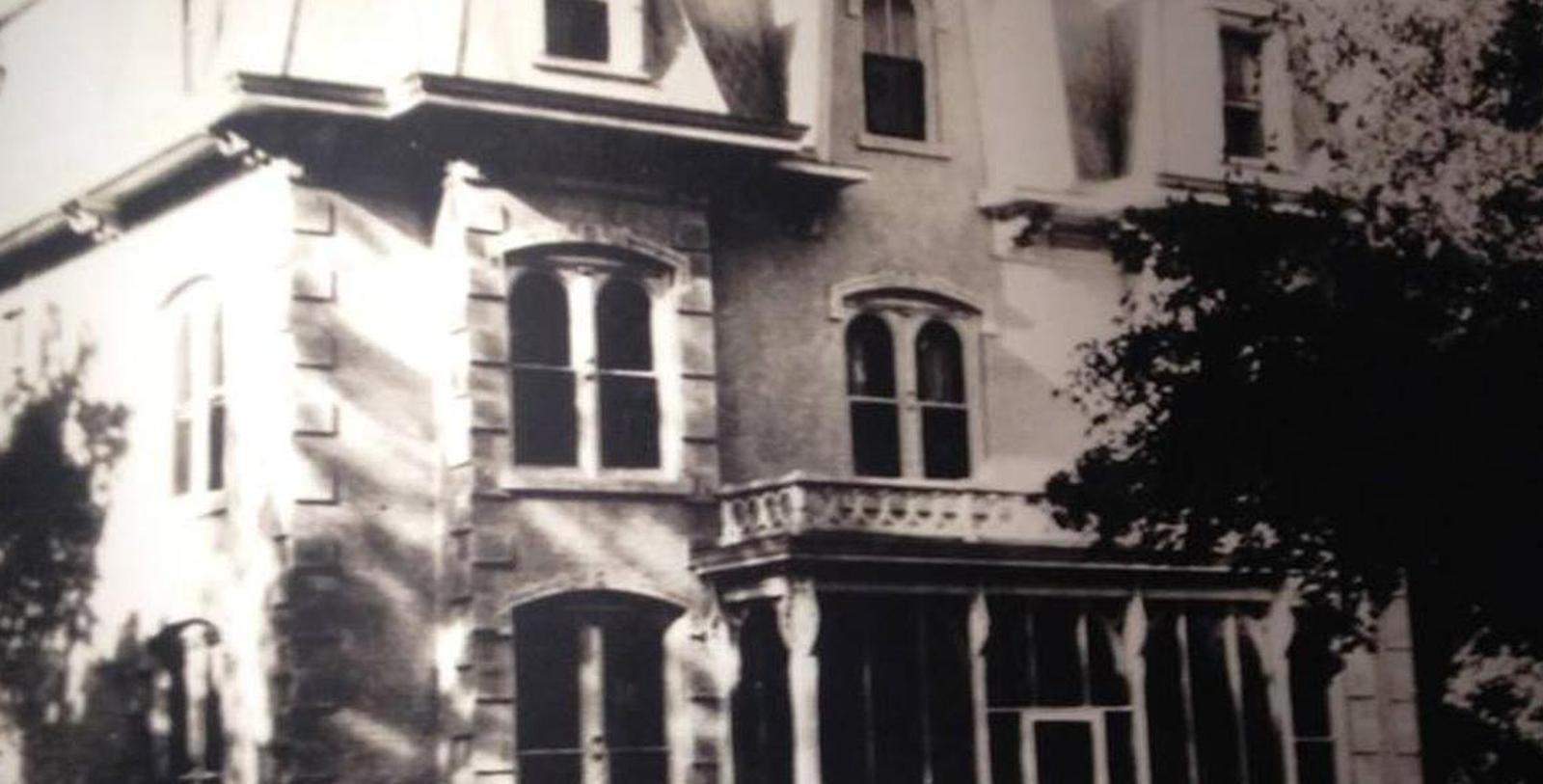This black and white photograph depicts a close-up view of a large, three-story early 20th-century building, likely made of stucco or cement, reminiscent of European architecture. The structure features numerous windows, including double-paned windows on the lower levels and arched, single-pane windows on the third floor, many of which are adorned with decorative stone accents. Central to the composition is an entryway porch supported by columns, above which sits a small balcony with a white fence. To the right foreground, the silhouette of a blossoming tree adds an organic contrast to the old, grand building. The intricate doorway design, shadows, and antique appearance evoke a sense of vintage elegance, enhancing the building's historic ambiance.